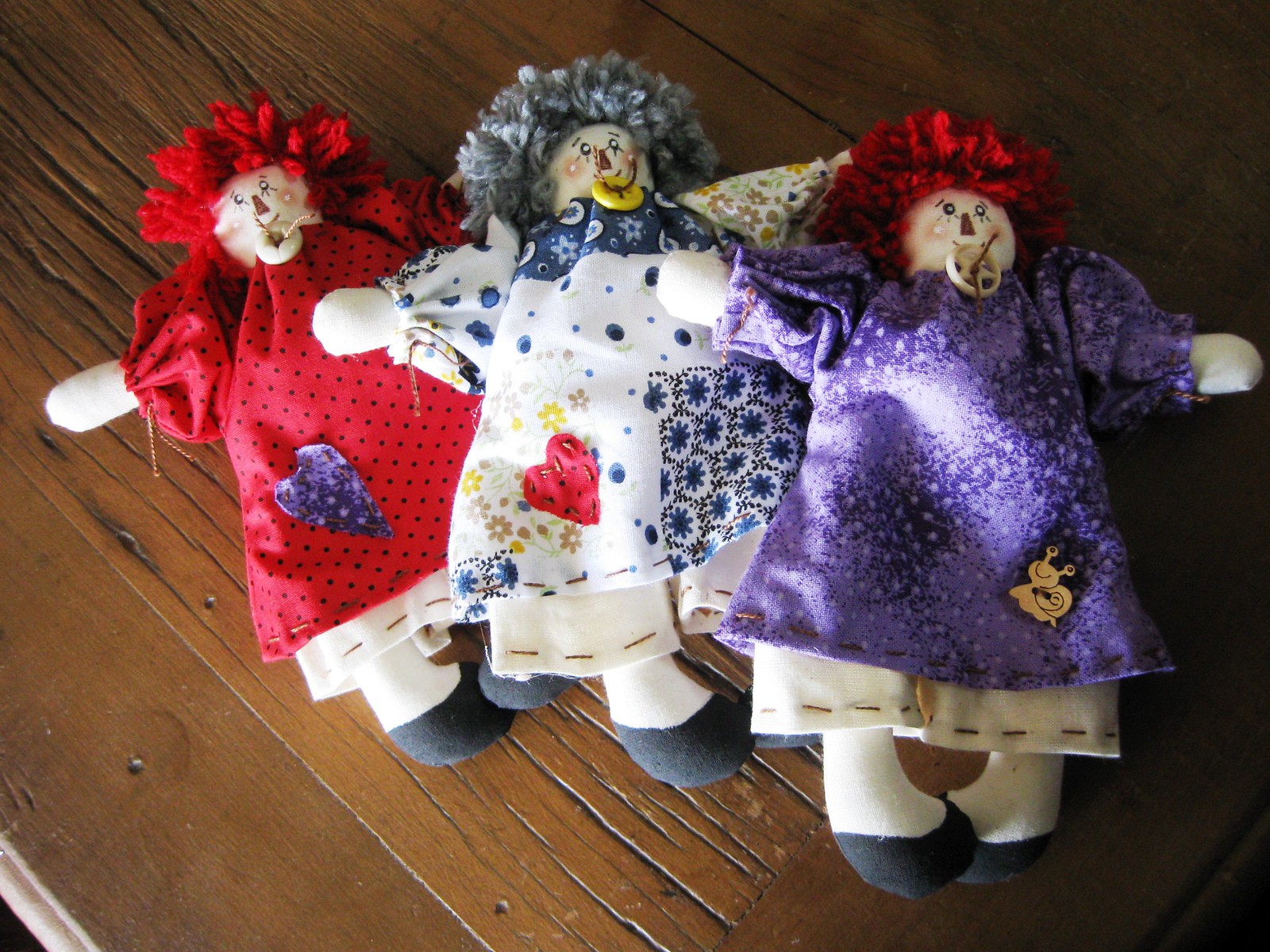The image depicts three handmade rag dolls lying flat on an old wooden tabletop, arranged in a partially stacked, partially fanned-out manner. These dolls are styled similarly to Raggedy Ann dolls and feature white fabric bodies with round heads, soft arms positioned to the sides, and legs that terminate in black fabric to suggest shoes. 

The leftmost doll is dressed in a red dress adorned with black polka dots and a purple heart sewn onto the bottom left corner of the hem. This doll has red yarn hair splayed out in all directions and a scarecrow-like face. It wears white pants with visible basting stitches around the ankle cuffs.

The middle doll's attire consists of a blue and white calico-patterned dress, accentuated with brown and yellow flower-like designs. A red heart with hand stitching is affixed to the left side of its dress. This doll sports grayish-blue yarn hair and, like the others, displays a scarecrow-like face. Below its neck, a yellow button can be seen.

The rightmost doll wears a purple dress with hand-stitched white accents. A snail patch embellishes the lower right side of her dress. This doll also features red yarn hair and a scarecrow-like face, along with a star-shaped white button at the collar. All three dolls are meticulously crafted from white cloth fabric, showcasing the detailed artistry through their unique decorations and stitching.